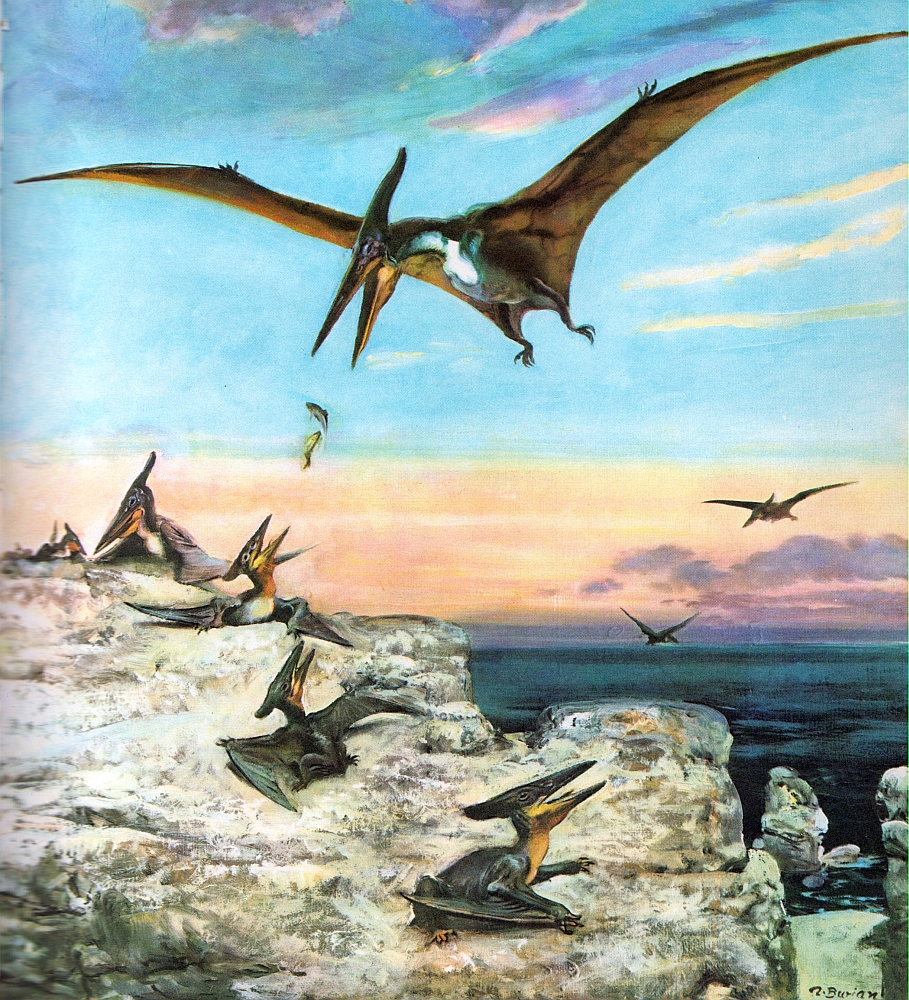The image depicts a detailed artwork of prehistoric times featuring various pterodactyls, the flying dinosaurs, focusing on a dramatic feeding scene. Dominating the top center, a large pterodactyl with outstretched, long wings, primarily light brown and green, appears to be gliding from right to left. This main pterodactyl, characterized by a sleek, vertical head with a protruding back and a large beak, is actively feeding its young, as evidenced by two fish being released from its mouth. Below, perched on a rocky cliffside, a smaller pterodactyl with its mouth open eagerly awaits the falling fish, ready to eat. 

In the bottom center, two additional young pterodactyls, sharing the same dark green and cream coloration, also sit with open mouths on the rocky terrain. Adding to the scene, a larger pterodactyl in the background to the left appears vigilant, possibly watching over another smaller pterodactyl nearby on the cliffside. The right side of the background features two more pterodactyls in flight.

The setting encompasses an ocean or lake with dark blue waters extending into the horizon, which is painted in shades of orange, red, and peach, indicative of either sunset or sunrise. The sky transitions into light blue, filled with clouds that range from purple to yellow, creating a vibrant backdrop for this prehistoric tableau.